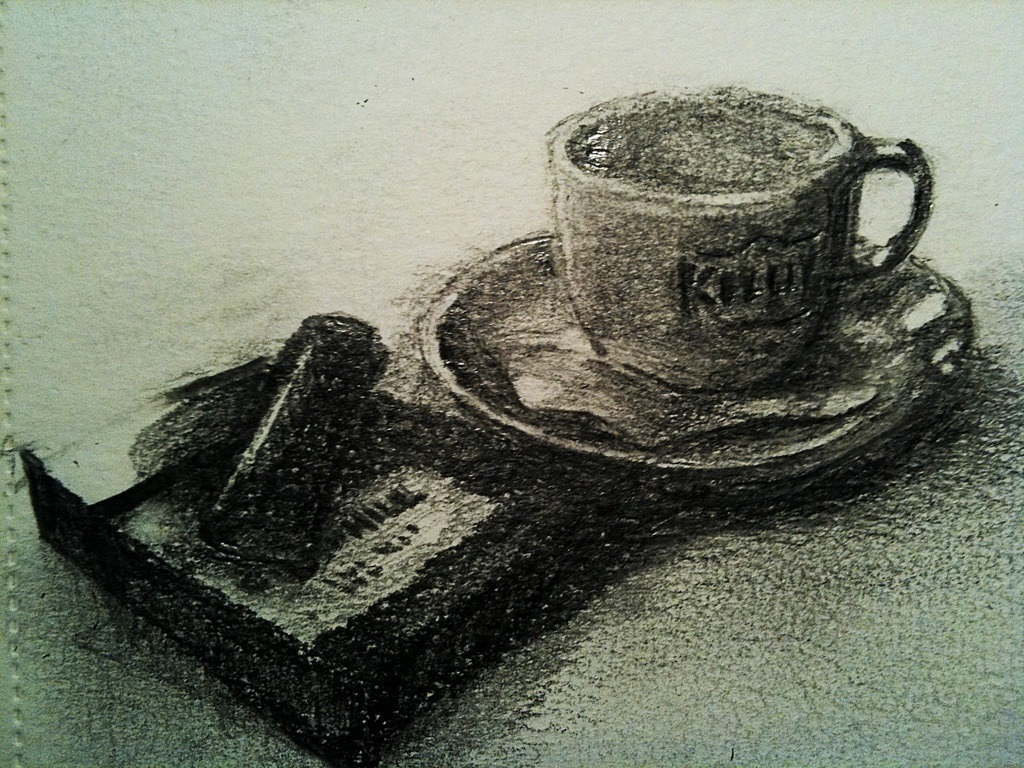A detailed charcoal drawing is depicted on a sheet of paper, evident from the left edge where perforations suggest it was torn from a spiral-bound sketch pad. Dominating the top right corner of the drawing, there is a coffee cup with a handle, intricately detailed with a design featuring letters and a shield on its front. The cup rests on a small saucer which seems to have a napkin placed between them. To the bottom left, a cigarette pack lies flat on its back, topped with a lighter oriented away from the viewer. The entire composition is skillfully rendered in shades of black, white, and grey, capturing the textures and nuances typical of charcoal medium.